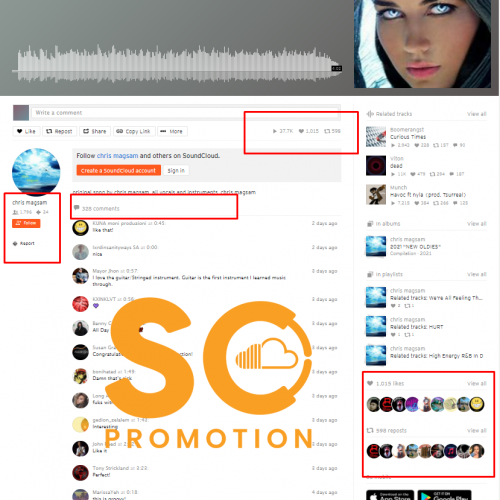In the image, a medium to darker gray banner is displayed at the top. On the right side of the banner, there's a partially seen image of a girl, showing only the area from her chin to just above her eyebrows. She has medium-toned skin, pink lips, a touch of blush, and striking icy blue eyes.

To the left side of the banner, there is a visual representation of a recording with volume levels indicated by up and down bars. Below this, there is a text bar that reads "Write a comment," followed by options for interaction: "Like," "Repost," "Share," "Copy Link," and "More."

Further down, a red square highlights some statistics: 37.7K likes, 1,015 hearts, and 598 shares. Beneath these statistics, there's text prompting users to "Follow Chris Maxim" (spelled out as C-H-R-I-S M-A-X-I-M) and others on SoundCloud. It also provides options to "Create a SoundCloud account" and "Sign in."

Towards the bottom, various circles containing images are displayed, and over the entire composition, there is a prominent text that reads "S-O Promotion."